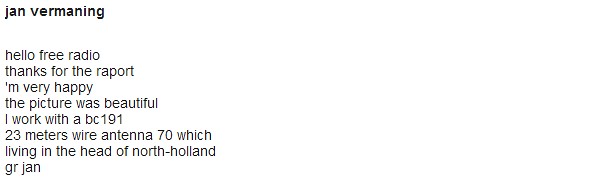The image features a white background with a block of text on the left side. At the top, in bold black text, is the name "Jan Bermanning." Below it, in regular black font, the text reads: "Hello, Free Radio. Thanks for the report. I'm very happy. The picture was beautiful. I work with a BC-191, 23 meters wire antenna, 70. Living in the head of North Holland, GR. Jan." This message appears to be a QSL response from Jan, a ham radio operator, expressing gratitude for a reception report and sharing details about his equipment and location in North Holland.